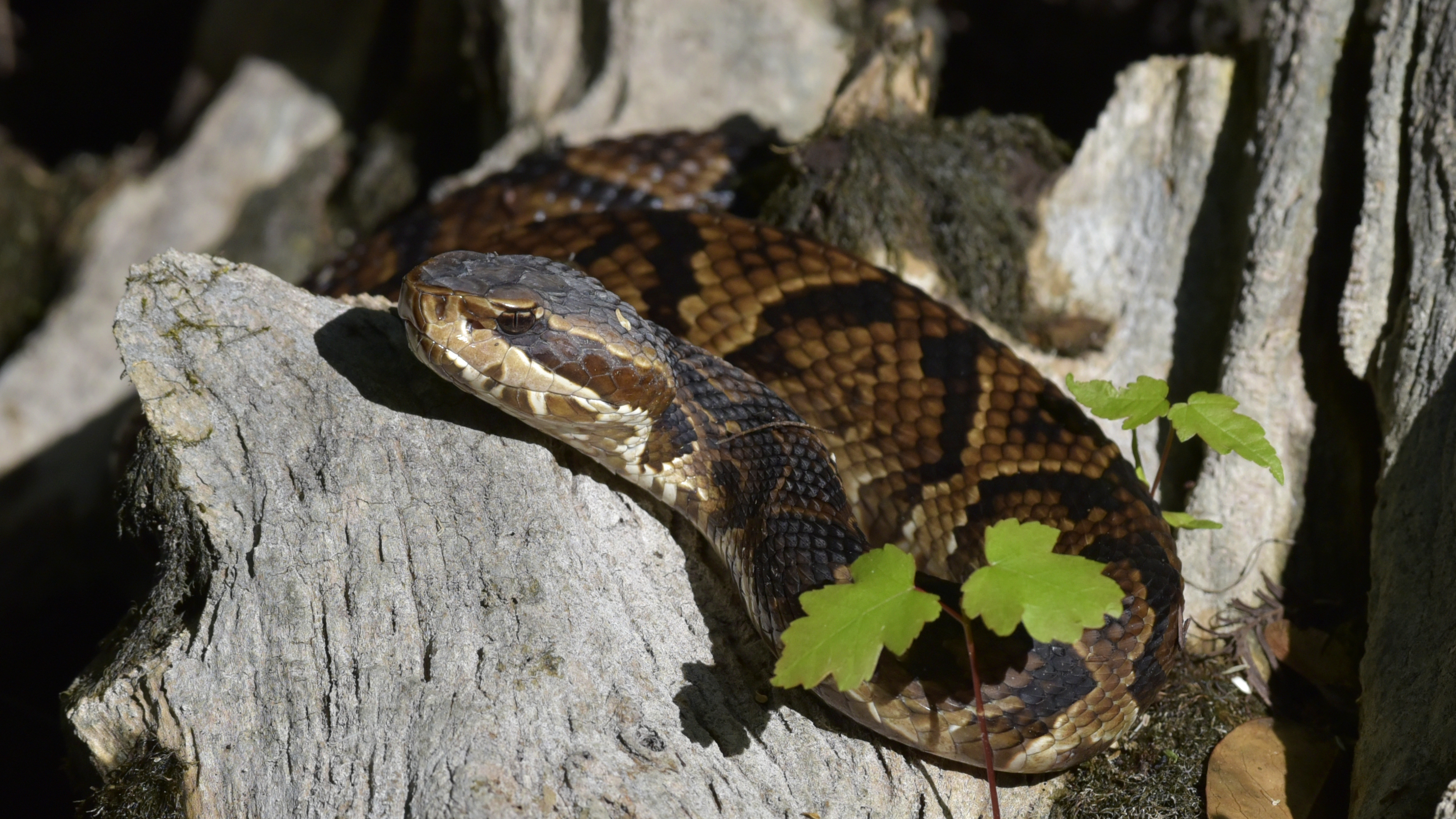This photograph features a brown-beige snake with distinctive black stripes, resting on a charcoal-colored tree branch or log in an outdoor setting. The scene is bathed in daylight, with sunlight illuminating the snake’s slightly lifted head, revealing a sliver of its eye. The snake, positioned centrally in the image, appears relaxed and uncoiled, almost as if it is sleeping with its eyes closed. Surrounding the snake are a few actively growing plants with bright green leaves and brownish-red stems, adding a splash of color against the gray and brown tones of the log and the surrounding foliage. Several trees are visible in the background. The image, formatted more in a widescreen dimension akin to a high-definition television, captures the tranquil moment in nature with a level of detail that highlights the textured patterns of the snake and the intricate growths on the log.